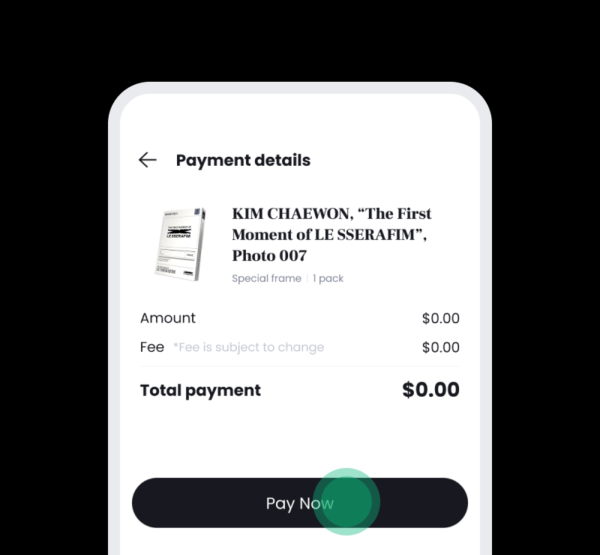The image features a rectangular layout with a black background, emphasizing the central focus: a partially visible smartphone screen superimposed over the dark backdrop. The phone, displaying its top half to two-thirds, has a distinct gray border framing the display. The screen itself shows a user interface with a white background.

At the top of the screen, there's a black left-pointing arrow, and adjacent to it, bold text that reads "Payment Details." Directly beneath this heading, on the left side, is a slightly out-of-focus image that appears to be silver-colored. Although indistinct, this image could be a photo, a book cover, or a game cover, featuring some black text.

To the right of this image, the text "Kim Chae Won" is written in capital letters, followed by the phrase "the first moment of Lee Seraphim" in quotes. Indicating a specific item, the text "Photo 007" is listed. Below this, smaller text states "Special Frame 1 Pack." On the left side below this description is the word "Amount" in dark text, paired with "$0.00" on the right. Further down, the word "Fee" appears with an asterisk, accompanied by the note "Fee is subject to change," and "$0.00" is listed next to it. The total payment is indicated as "$0.00."

At the bottom of the smartphone screen, there is a prominent black button with the text "Pay Now," inviting the user to proceed with the transaction.